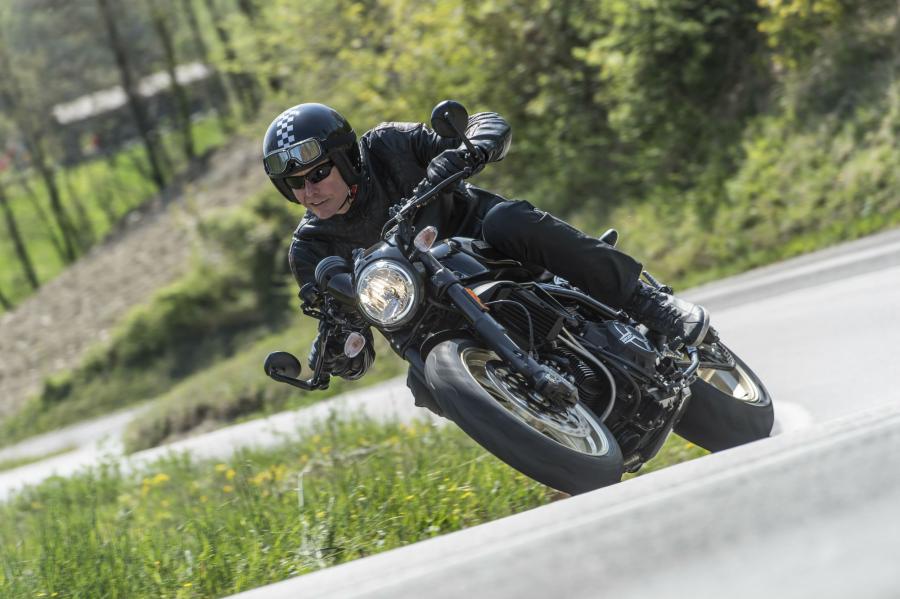This detailed photograph captures a motorcyclist deeply leaned into a sharp corner on a windy asphalt road. The rider, clad entirely in black motorcycle gear including a black helmet adorned with a checkered pattern and striped design, black leather jacket, black leather gloves, black jeans, and black boots, is tilted at an almost 45-degree angle to the road. The motorcyclist, who is Caucasian and wearing black sunglasses, is gripping the mostly all-black motorcycle, distinguished by its prominent headlight. The helmet also has goggles attached, although they are not in use, as the man appears to be smoking. The background is rich with natural elements, featuring green grass, a mix of shrubs, and a dense array of trees with visible brown trunks both to the left and right of the scene. Notably, there is a brown wooden structure peeking out from the far left side, adding a rustic touch to the lush scenery. The close proximity of the man and his motorcycle to the camera emphasizes the dynamic movement and steep angle of the turn.